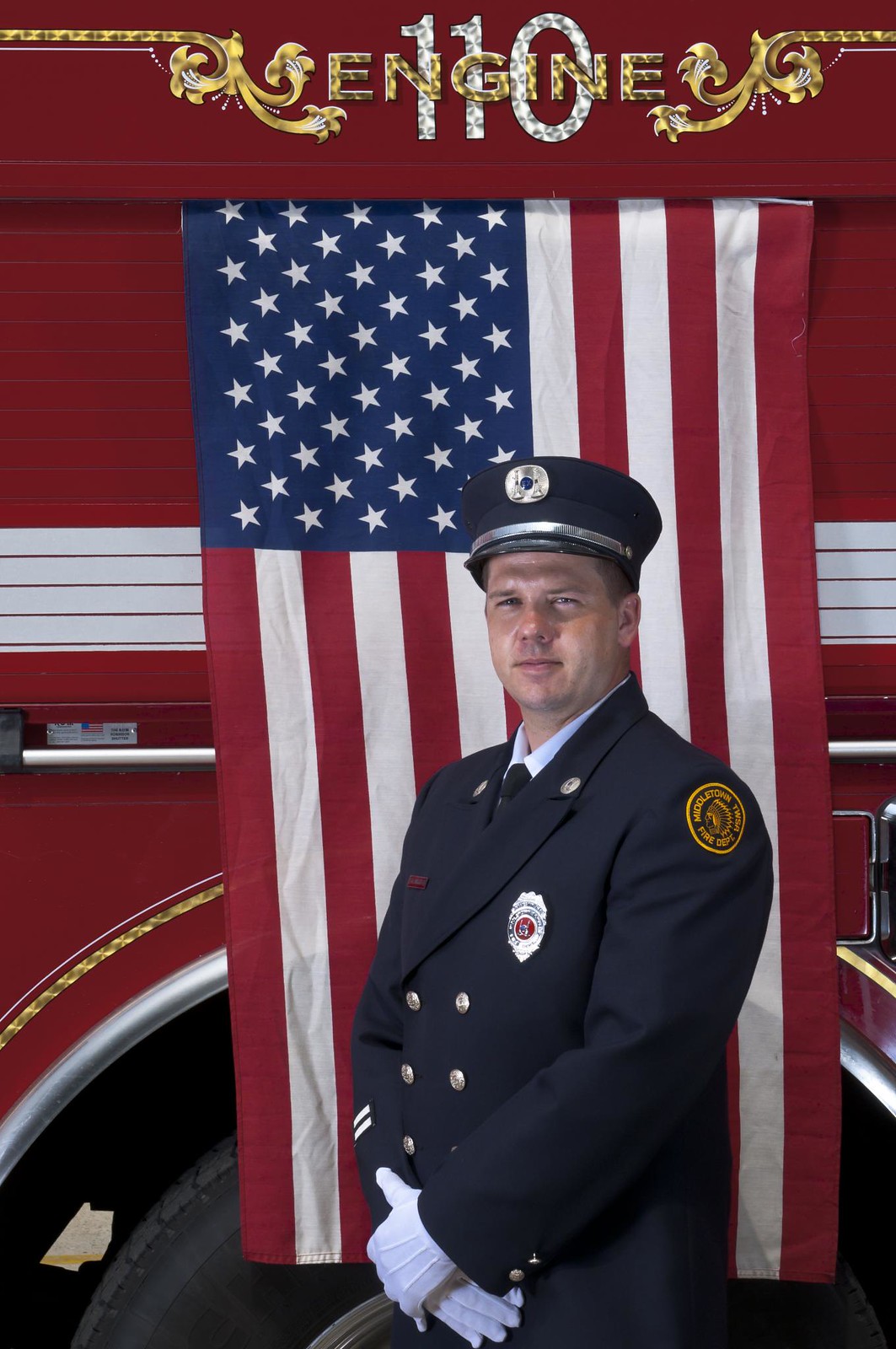The image features a formal portrait of a Caucasian male firefighter, dressed in an immaculate formal dress uniform. He is wearing a dark blue coat adorned with a shiny fire badge on the front and a circular gold logo on his left shoulder, which reads "Middleton Fire Department" with additional text encircling an inner image. Beneath his jacket, he sports a crisp collared shirt and a tie, paired with pristine white gloves. His arms are crossed at his waist in a three-quarter view stance, facing towards the camera with a neutral expression. On his head, he wears a cap reminiscent of a police officer's, featuring a short brim. He stands in front of an American flag draped from a fire engine, which is elaborately decorated with gold and silver designs. The fire engine prominently displays "Engine 110" with the word "Engine" in patterned gold letters above the patterned silver numerals "110." The picture is brightly lit, likely by natural light, making the details clear and vivid.